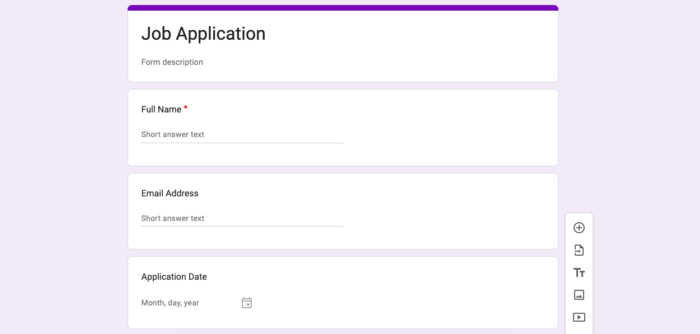The screenshot showcases a Google Forms application dedicated to a job application process, set against a background featuring a soft gradient of light purple, pink, and lilac hues. The form's design is accentuated by a prominent dark purple bar at the top, adding a touch of elegance to the interface. 

On the right side of the form are various icons, likely offering customization options or functionalities for filling out the application. The form itself is streamlined and user-friendly, divided into four primary sections, each with black text on a white background.

1. At the top is the main heading, "Job Application," accompanied by a space for the form description.
2. Below that, the form prompts the user to enter their "Full Name," highlighted by a red asterisk indicating a mandatory field, followed by a short answer text box for input.
3. The third section requests the applicant's "E-mail Address," again with a corresponding short answer text box for entry.
4. Finally, the form asks for the "Application Date," where applicants can select the date using a convenient month, day, and year format, with an option to choose the date from a calendar widget to the right.

The overall simplicity and minimalistic text imply that this screenshot is likely taken from the creator's perspective, as they configure the form for future applicants to complete.